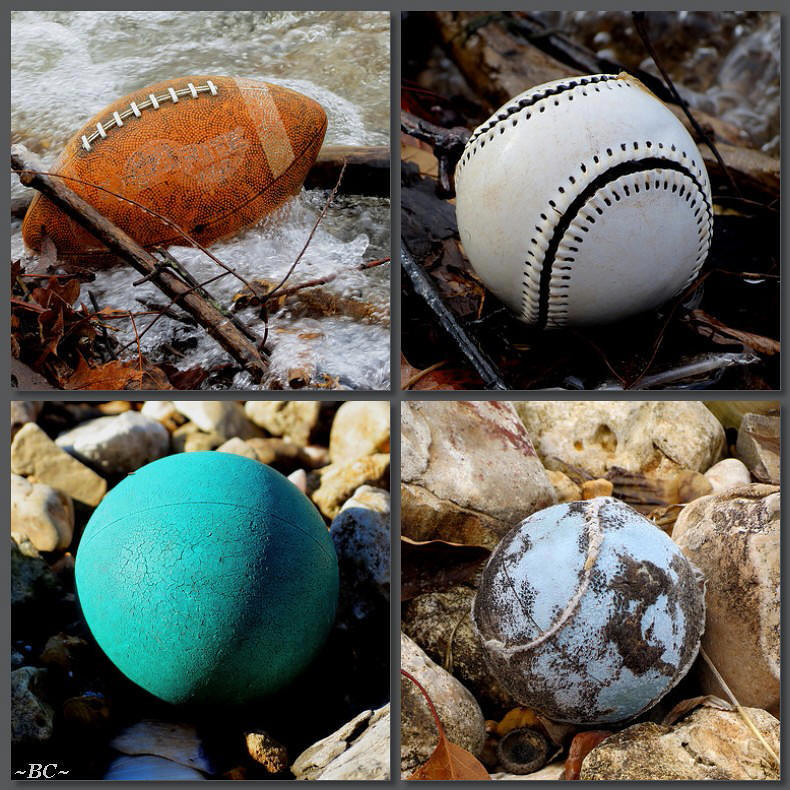The image consists of a photo grid with four equally-sized, smaller photos arranged in a 2x2 layout. 

- The upper left photo shows an American football, noticeably worn and saturated with a deep orange hue, floating in a fast-moving river. The water is strewn with sticks and leaves, and the football's logo is faded beyond recognition.
  
- The upper right photo features a white baseball with black stitching. The baseball, although somewhat worn, lies amidst a jumble of sticks and leaves, captured in a close-up shot.
  
- The bottom left photo displays a blue rubber ball perched on a pile of blurred rocks. The ball exhibits visible signs of cracking, likely due to exposure to the sun or extensive use.

- The bottom right photo captures a very weathered blue baseball with peeling cloth stitching. It rests among large, natural-colored rocks, appearing as if a layer of the leather cover has been stripped away, revealing the interior.

The overall composition reveals the effects of nature and time on different types of sports balls placed in various outdoor environments.